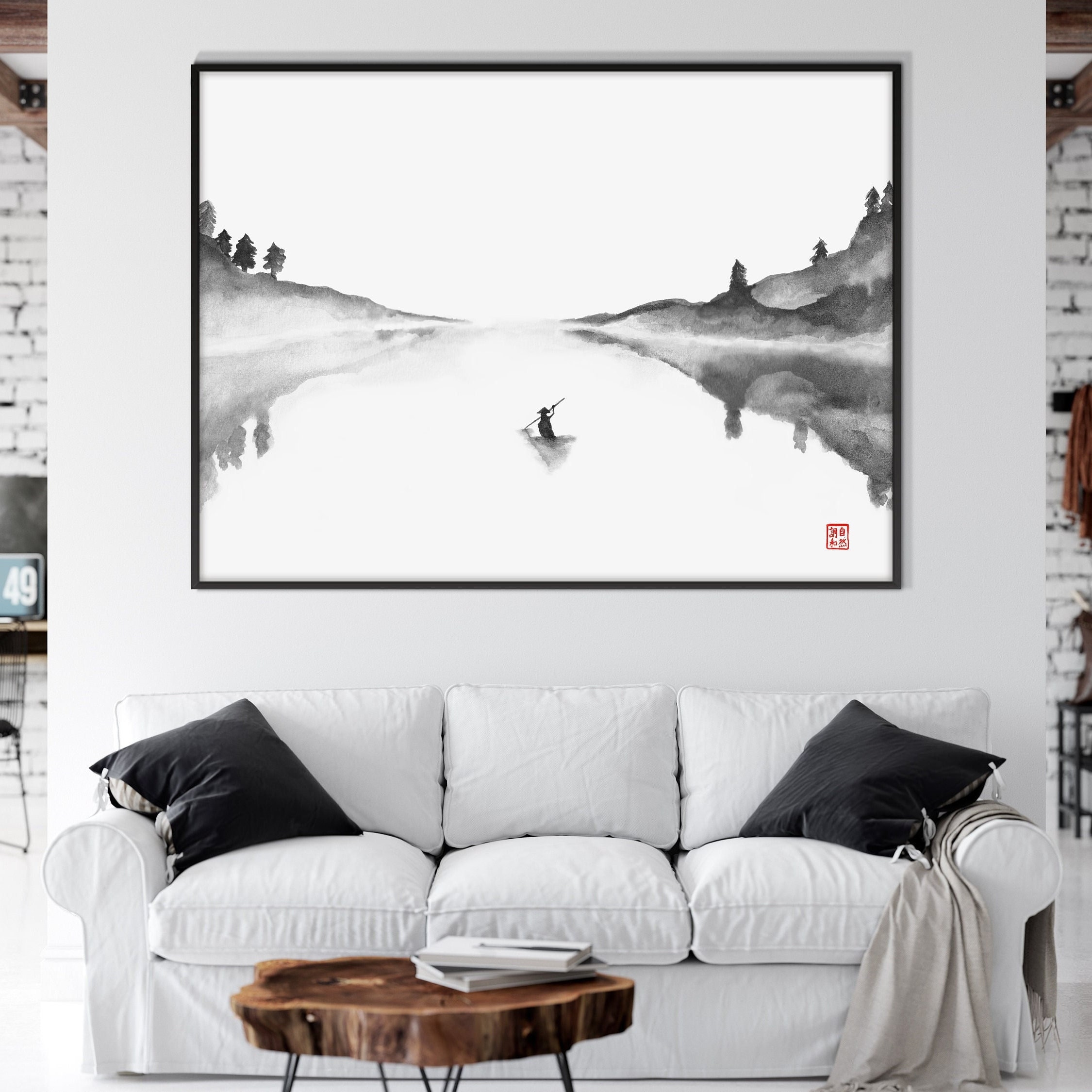The photograph captures the tranquil ambiance of a minimalist living room. The focal point is an expansive painting styled in traditional Japanese watercolor, predominantly black and white, depicting a figure paddling down a river, flanked by subtle gray landscapes, with a red Chinese name mark at the bottom right. This artwork hangs on a striking light gray wall, which contrasts with the pristine white slipcovered couch below. The couch, adorned with two black pillows—one at each end—and a beige-gray blanket draped over its right arm, serves as a harmonious base. In the foreground, a rustic coffee table made from a large wood slice sits on spindly metal legs, bearing a few neatly stacked white books. The sparse decor and natural elements, including glimpses of white brick framing the scene, suggest a room defined by elegant simplicity and serene modernity.